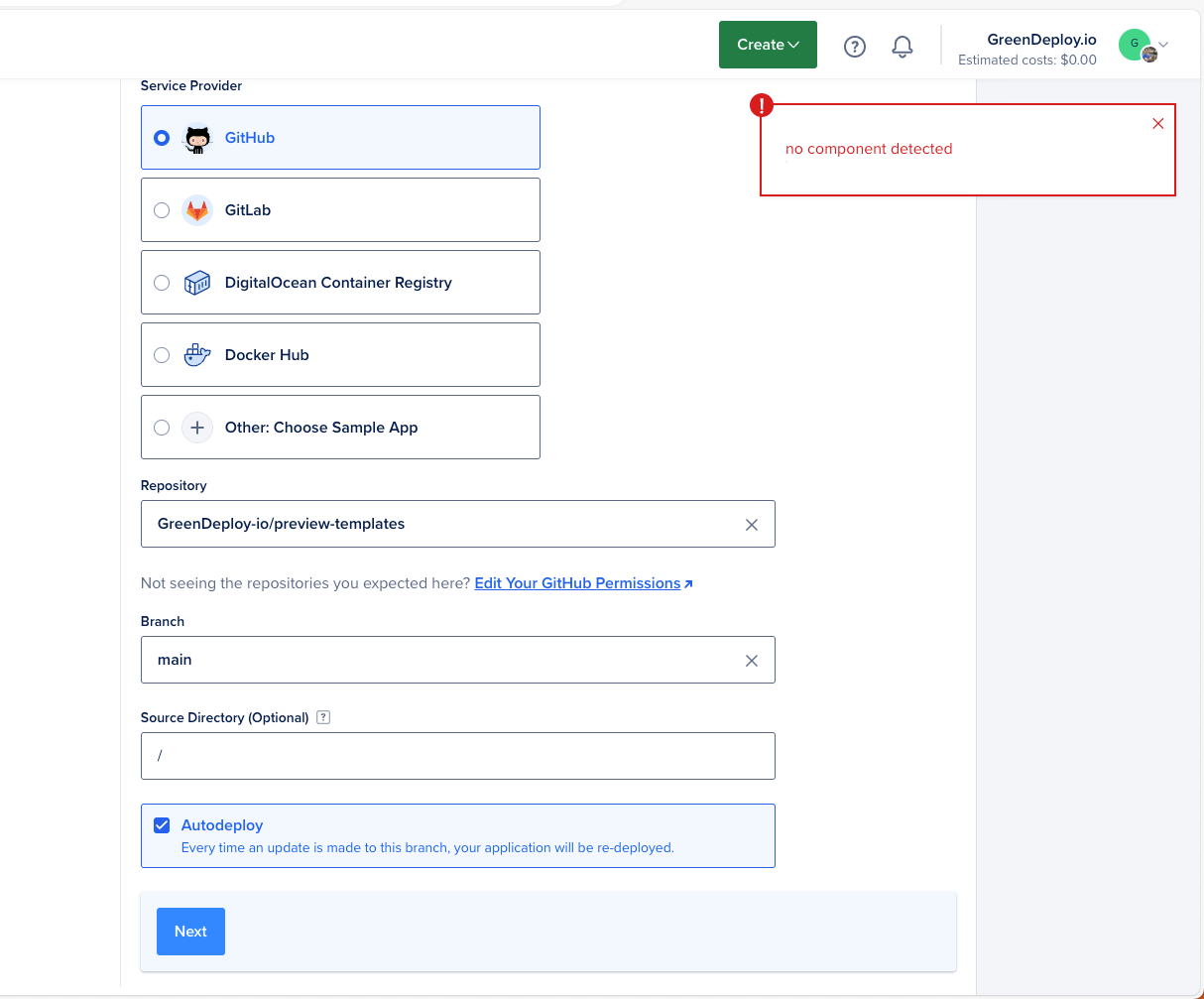Here is a detailed and cleaned-up caption for the image:

---

This is a screenshot of a web page for an application or program interface. At the top, there is a white navigation bar. On the right-hand side of this bar, there is a green button labeled "Create" in white text, accompanied by a drop-down arrow. Following this button, there is a circular icon with a question mark, a bell icon, and text reading "screen deploy.io" on the far right.

Beneath the navigation bar, the text "Estimated Costs: $0.00" is displayed next to a green circle with the letter 'G' inside it, which contains a smaller circle and a drop-down arrow.

Below this section, a large red box is presented with the message "No component detected" featuring an exclamation point and an 'X' icon on the right side.

On the left-hand side of the page, a list of service providers is available for selection, each within a large rectangle. The options include:
1. GitHub (selected, displaying the GitHub logo and the text "GitHub"),
2. GitLab,
3. DigitalOcean Container Registry,
4. Docker Hub,
5. Plus another option labeled "Choose Sample App."

Further down the page, a drop-down menu labeled "Repository" is shown, displaying the path "green deploy-io/preview/templates." There is a prompt that reads, "Not seeing the repositories you expected? Edit your GitHub permissions." Additional fields include "Branch" (set to "main"), "Source Directory" (optional), and an "Auto Deploy" toggle.

At the very bottom on the left-hand side, a blue button with white text labeled "Next" is visible.

---

This description includes all elements and details originally mentioned, restructured into a coherent and detailed caption.